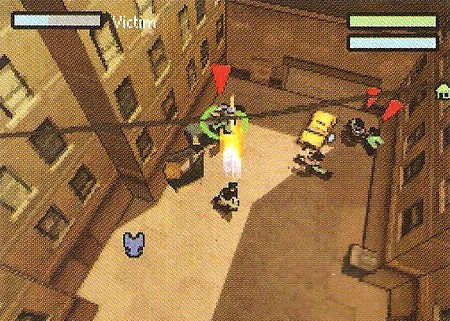The on-screen gameplay image showcases several characters in a dynamic urban setting. At the top of the screen, the word "victim" is prominently displayed. Below this, a health bar, divided into light and pinkish segments, indicates the remaining life force of a character. In the upper-right corner, two parallel rectangular bars are visible—one yellow and the other white. The scene is set against a backdrop of tall, brown buildings that feature numerous windows and surround a brown, concrete ground. Four characters are scattered throughout this urban environment, poised for interaction within the gameplay.